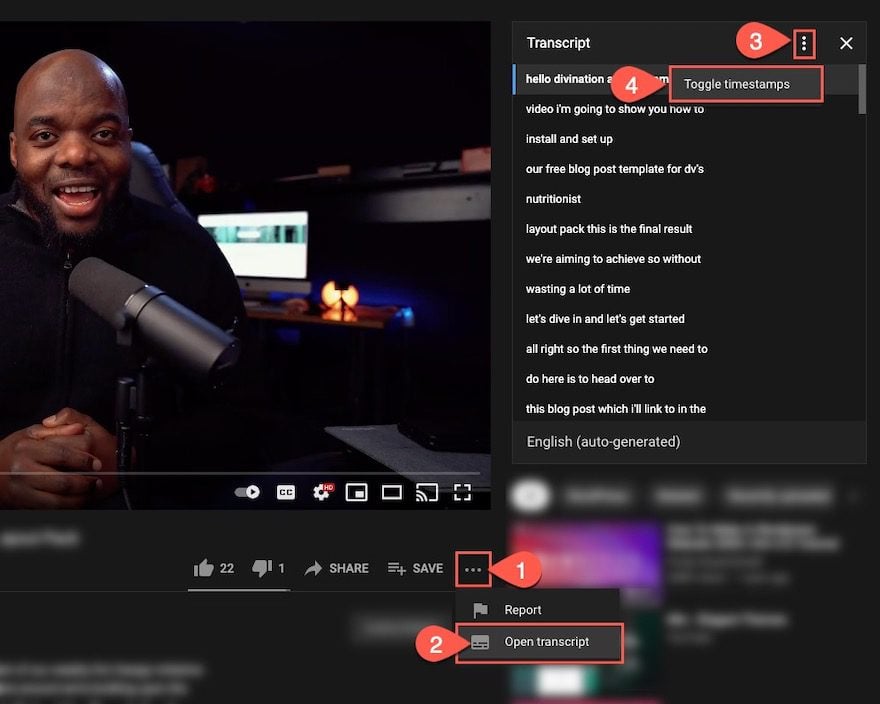The image is a detailed screenshot from a YouTube live stream on a desktop. The snapshot captures the right half of the webpage, predominantly featuring the chat section, but the chat is not visible as the transcription feature has been activated. The image includes step-by-step annotations, guiding the viewer on how to access and use the transcription tool. 

1. **First Step:** Click on the three vertical dots located at the bottom right of the video player.
2. **Second Step:** A drop-down menu appears; select the 'Open Transcript' option.
3. **Third Step:** Once the transcript panel is open, click on the three dots within the transcript.
4. **Fourth Step:** Another drop-down menu appears, offering the 'Toggle Timestamps' option among other settings.

The auto-generated captions from the video are displayed in the transcript panel. Additionally, the live stream has garnered 22 likes and 1 dislike, emphasizing the community's mostly positive reception. The screenshot serves as a tutorial for users looking to utilize YouTube's transcription and timestamp features.